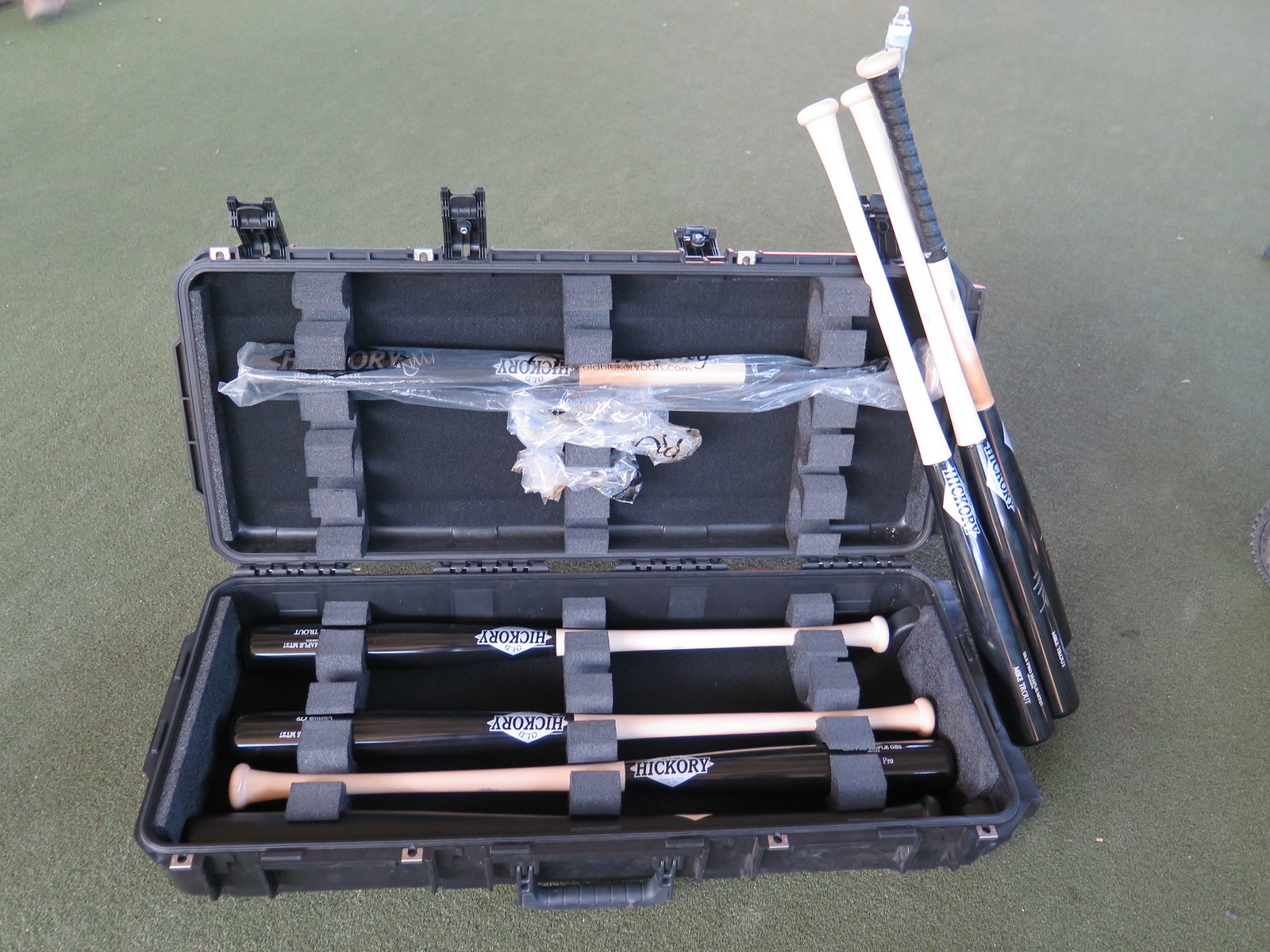The image is a color photograph taken outdoors during the day, featuring an open black sports case, often mistaken for a gun case, resting on what appears to be a light grayish-green astroturf or concrete surface. The open case reveals brand-new hickory baseball bats neatly arranged within gray foam separators. 

Inside the case, three identical bats lie horizontally at the bottom, each showcasing a natural wood base and a black top adorned with a diamond logo and the word "Hickory" written in bold. Additionally, one bat, still wrapped in plastic, is positioned diagonally on the upper portion of the case, indicating space for more bats. 

To the right of the case, three more bats stand upright, leaning against the case. All the bats appear to have a similar design, with the notable exception of one bat featuring tape wrapped around its handle.

The entire setup sits against a flat, grayish-green background with no visible text or markings other than the labels on the bats, perfectly capturing the organized display and pristine condition of the hickory bats within the case.